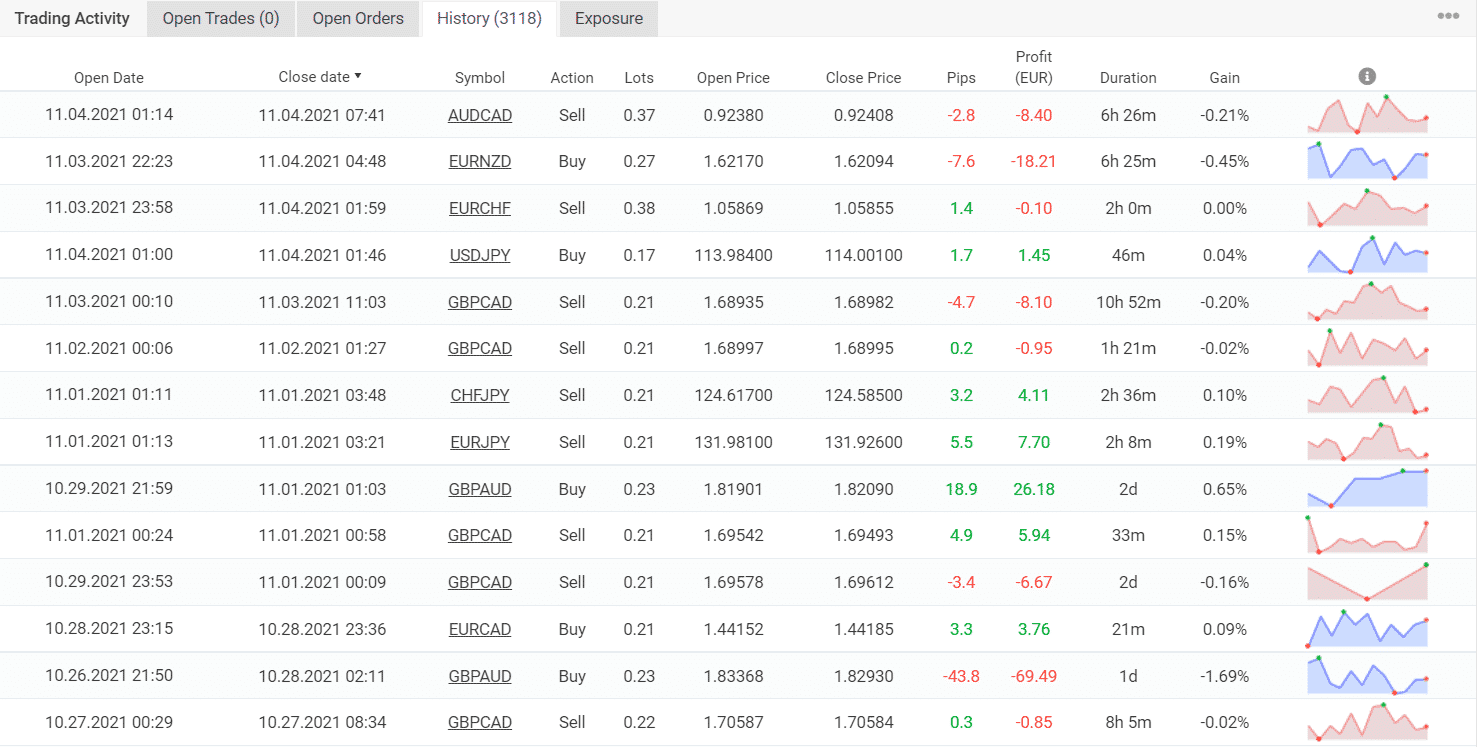The image features a detailed chart documenting trading activity, organized under multiple tabs located at the top left of the display. These tabs include "Trading Activity," "Open Trades (0)," "Open Orders," and a highlighted "History (3,118)," along with "Exposure," all presented in gray text or boxes.

The main body of the chart is segmented into several columns: "Open Date," "Close Date," "Symbol," "Action," "Lots," "Open Price," "Close Price," "Pips," "Profit (EUR)," "Duration," "Gain," and an icon resembling an eye within a gray circle, possibly denoting visibility or insight.

Beneath these column headers, the chart lists 14 different trading entries. Each entry details specific trade information including:
- The dates when trades were opened and closed.
- The trading symbol associated with the item.
- The action taken, whether "Buy" or "Sell."
- Quantities in "Lots."
- Opening and closing prices.
- The amount of "Pips" gained or lost.
- Profit figures, shown in either red (loss) or green (gain).
- The duration of the trade.
- The percentage "Gain."
- A small graphical representation at the end, either red or blue, perhaps indicating trends or outcomes.

The comprehensive layout captures a snapshot of comprehensive trading records, presented with clarity and precision.